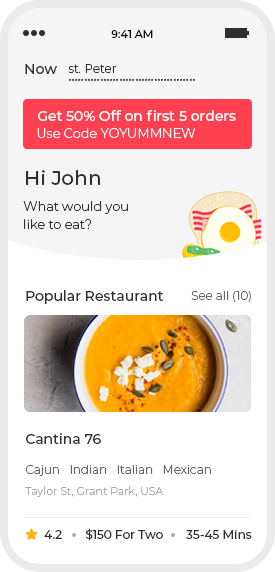This image showcases a smartphone layout screen, likely from a food delivery app. The top left corner features three horizontal black bars, indicating a menu or navigation icon. Centrally positioned at the top of the screen is the time, 9:41 AM. To the right, a battery icon is displayed, fully charged.

Beneath the top bar, a header reads "St. Peter," with the text stylized as "St." in lowercase and "Peter" with a capital P. Underneath this title is a string of dots or very small text. The background for this top section is a light gray color.

Prominently displayed below the header is a red box containing a special offer: "Get 50% off on your first five orders. Use code: YOUUMMAW." All the text within this box is white, with "Get 50% off on your first five orders" in slightly bolder font.

Further down, the message "Hi, John, what would you like to eat?" greets the user. Accompanying this text, on the right side, is an image of a breakfast consisting of bacon, eggs, and toast.

The screen transitions with a complex break, with the upper section of the background in gray and the lower part in white. The next section introduces a "Popular Restaurant," displayed in black text, followed by "CO" in smaller gray text.

Additionally, the screen provides details about a restaurant named "Cartina," associated with the number 76, and an image resembling a squash soup. The cuisine options listed include Cajun, Indian, Italian, and Mexican, alongside the locations Taylor-Oakley and Grand Park, USA. The restaurant is rated 4.2 stars and offers an estimated price of $150 for two people, with an expected delivery time between 35-45 minutes.